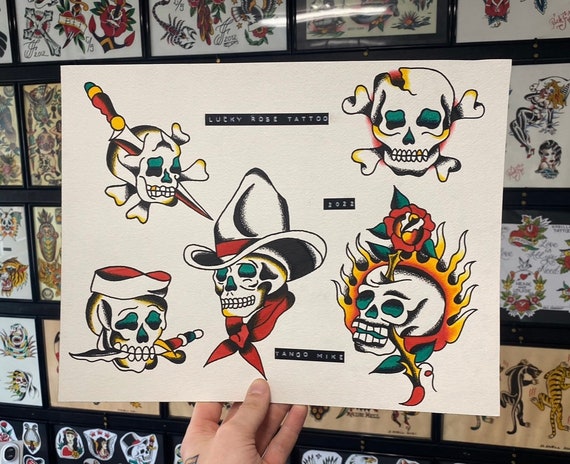A color photograph captures a moment inside a tattoo parlor. Dominating the image is a white piece of paper held by a left hand, thumb in front and fingers behind, filled with various tattoo designs centered on skull motifs. In the upper left corner, a skull and crossbones feature a knife pierced through it. The lower left depicts a skull gripping a knife between its teeth. Centrally, a skull is adorned with a large cowboy hat and a red kerchief. To the right, a menacing flaming skull contrasts with a simple skull and crossbones in the upper right. The background reveals a black wall adorned with additional tattoo artwork, though they are less prominent. Overlaying the scene, text on black tape reads "Tango Mike and Lucky Rose Tattoo 2022."